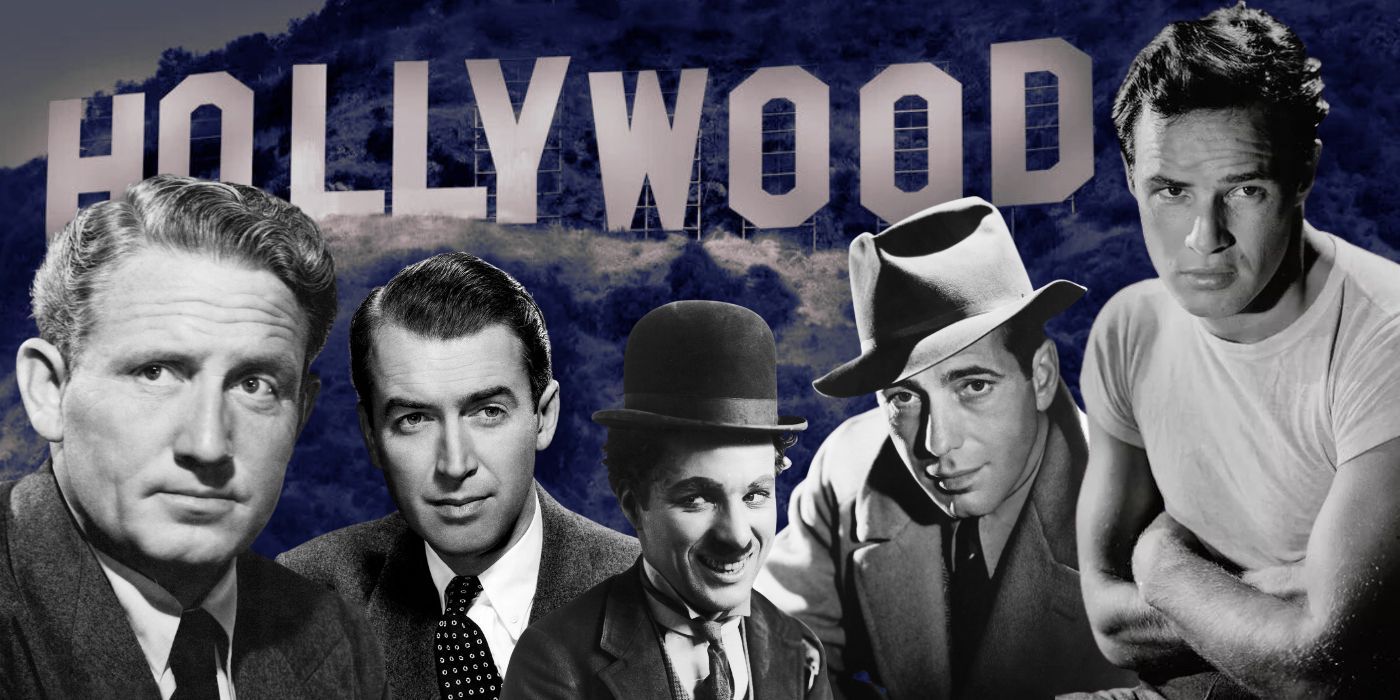Promotional Image: Historic Hollywood Icons Against the Iconic Hollywood Sign

This promotional image captures the timeless allure of Hollywood, California, showcasing the famous Hollywood sign atop the grassy hill. The sky peeks through in the upper left corner, adding a touch of serenity to the scene. Dominating the foreground are black-and-white headshots of five legendary male actors, assembled in a row, reminiscent of a Hollywood-themed Mount Rushmore. From left to right, the celebrated faces of Marlon Brando, Humphrey Bogart, Charlie Chaplin, Jimmy Stewart, and Spencer Tracy—formerly married to Katherine Hepburn—are prominently featured. These classic Hollywood icons are set against a subtly faded hillside, with the Hollywood sign imbued with a faint pink hue, adding a nostalgic charm and highlighting their collective impact on film history.